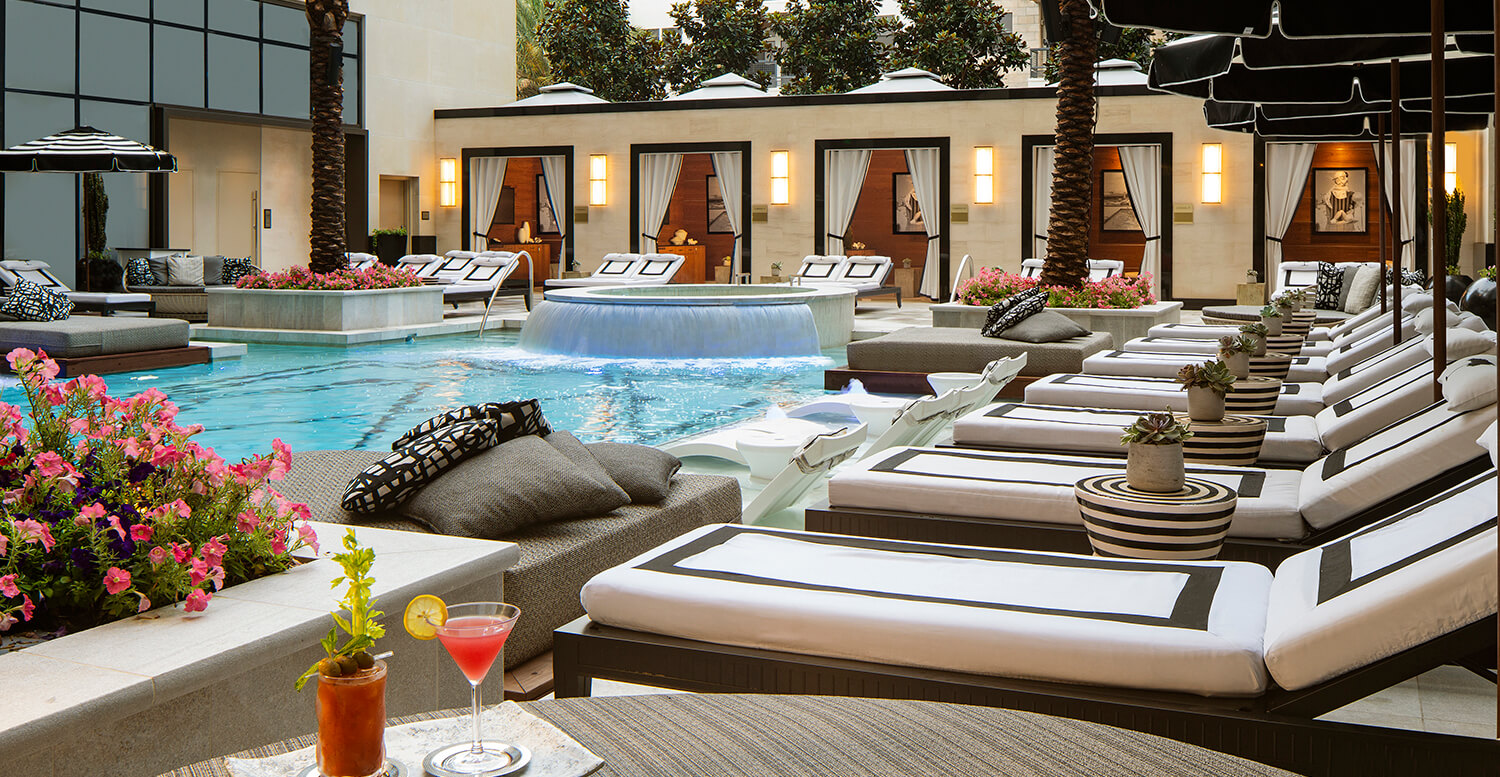This is a color photograph of a luxurious outdoor swimming pool area, likely part of an upscale hotel or resort. The pool, with its clear turquoise water, is surrounded by sleek black-and-white lounge chairs, each shaded by a black umbrella. Circular tables beside the loungers hold potted succulents. In the foreground, a white towel is draped over a table, holding two vibrant cocktails: a Bloody Mary and a pink martini with a lemon wedge. The pool area features a circular hot tub with water flowing into the main pool. Elegant cabanas line the side, each with curtains for privacy, and adorned with artwork and TVs inside. Two palm trees add a tropical touch to the scene. A larger building with glass windows is partially visible to the left, suggesting additional amenities or accommodations. Rows of pink flowers and the meticulous design contribute to the overall opulent and inviting atmosphere.